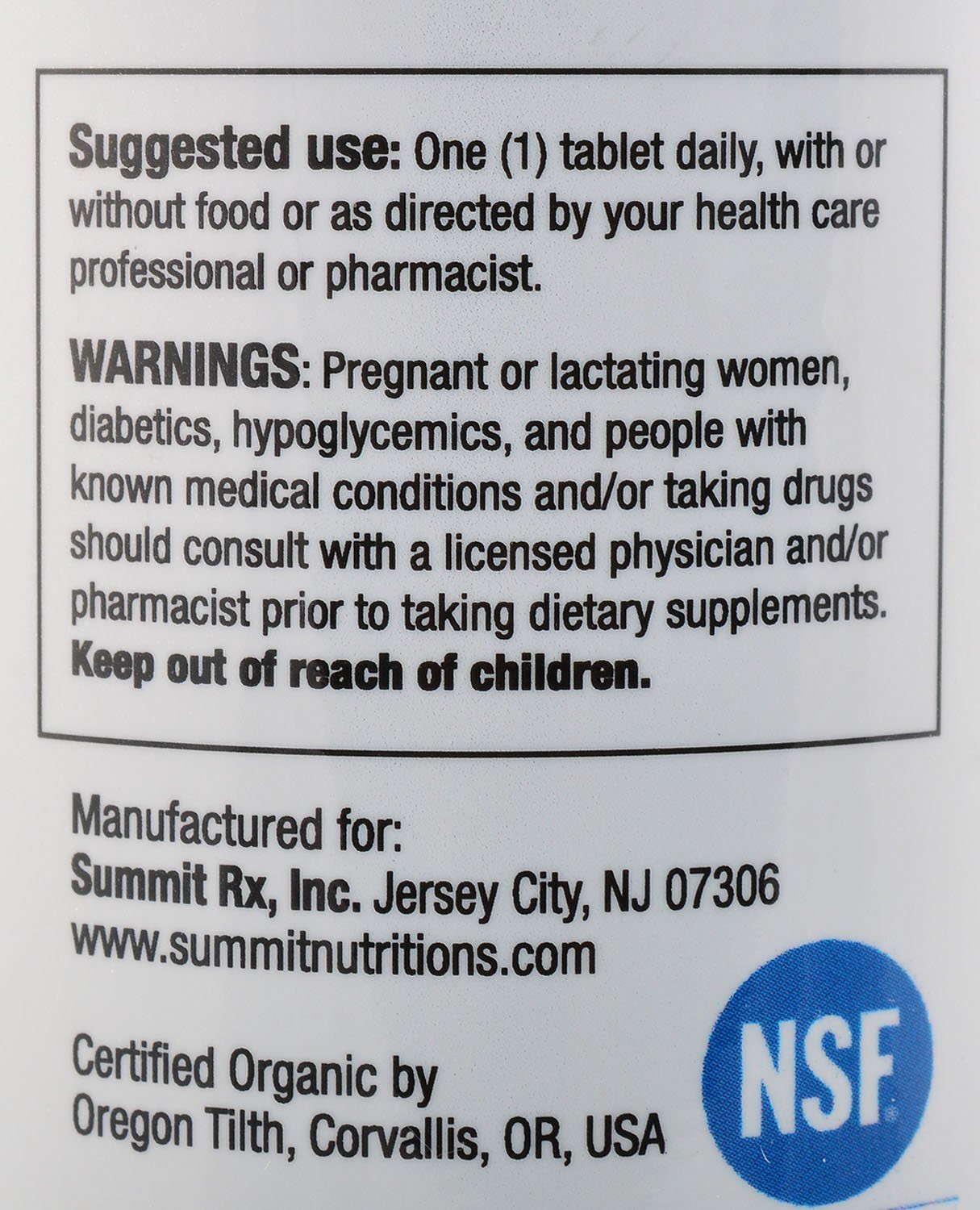A close-up photograph of a product label reveals detailed instructions and warnings. The label reads: "Suggested Use: One tablet daily with or without food, or as directed by your healthcare professional or pharmacist. Warnings: Pregnant or lactating women, diabetics, hypoglycemics, and individuals with known medical conditions and/or taking medications should consult with a licensed physician and/or pharmacist before using dietary supplements. Keep out of reach of children." The label indicates that the product is manufactured for Summit Rx, Inc., located in Jersey City, New Jersey, with a zip code of 07306. The company's website is provided as www.summitnutritions.com. The label also mentions certification by Oregon Tilth, based in Corvallis, Oregon, USA, and displays a blue seal with the letters "NSF" in white, denoting an NSF certification. The text curves slightly, suggesting that the label is affixed to a cylindrical container or bottle.